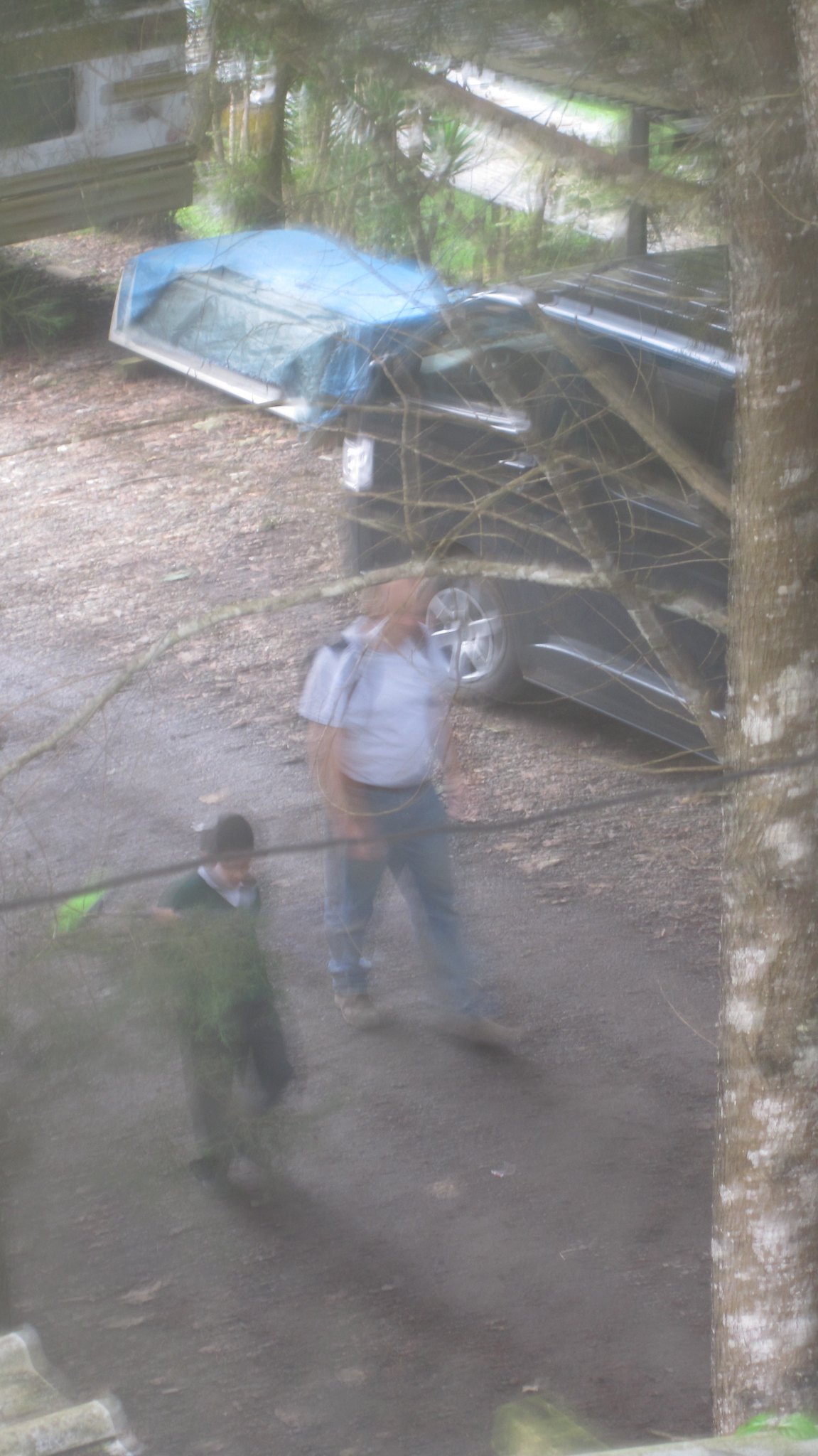In the photograph, two men are walking on a muddy, compacted road, surrounded by a forested area with numerous trees. The image is a bit blurry, making it difficult to discern their facial features clearly. One man is dressed in a dark suit, which appears black or navy blue, paired with brown boots. The other man wears blue jeans, a light-colored blue shirt, and brown shoes while sporting a bald head. Behind them to the right, there is a dark blue minivan, complemented by another vehicle partially covered by a light blue tarp. In the background, a white bus is visible, and the sky above is a medium light blue. The scene is further shaded by the dense foliage of the surrounding trees.